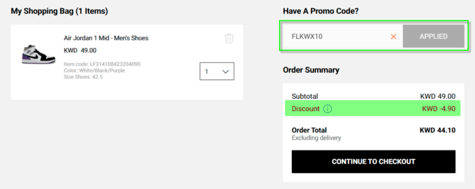This image displays a website interface showcasing an online shopping bag. In the top left corner, the text "My Shopping Bag, 1 Item" indicates the contents of the bag. The main focus is an image of Air Jordan 1 Mid Men's Shoes prominently displayed within a white rectangle. Next to the image, the product name "Air Jordan 1 Mid Men's Shoes" is clearly stated alongside its price, "KWD $49." Below the price, there is a trash bin icon, allowing users to remove the item. Adjacent to the trash bin is a small rectangle featuring a quantity indicator and an arrow for adjusting the number of items.

On the right-hand side of the image, the phrase "Have a promo code?" is presented in bold black letters. Below this, a green rectangle provides a field for entering a promo code, and within this field, a black rectangle with the word "Applied" signifies that a promo code has been used.

Further down, the order summary is displayed: the subtotal is listed as "KWD $49," followed by a discount shown in a green rectangle as "KWD -$44.90," resulting in an order total of "KWD $4.10." At the bottom, a prominent black rectangle with white text reads "Continue to Check Out," prompting the user to proceed with their purchase completion.